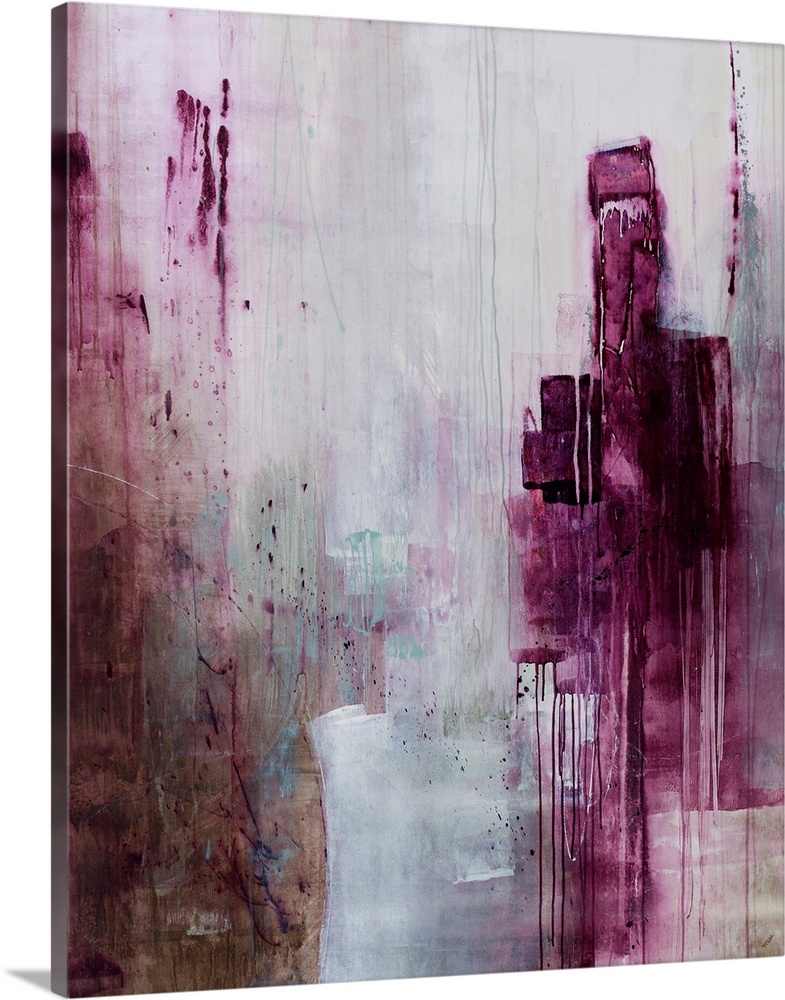This image features a detailed, abstract canvas painting with a portrait orientation. It is slightly tilted to the bottom left, showcasing a range of bold and muted tones. Predominantly, the piece is covered in a gray paint with thick, plummy purple brushstrokes that create a dynamic flow of color. Notably, on the right side, these dark purple shapes are interrupted by streaks of water that dribble down the canvas. In the center, vertical brush strokes of white and grayish tones create the illusion of a ghostly city skyline or building, adding a spectral quality to the artwork. The painting is further textured with random purple spots and a brownish section at the bottom left, enhancing its unfinished and weathered appearance. Additionally, bluish hues near the center and dark red splotches at the top left contribute to the overall complexity, with spatters and dribbles interspersed throughout. This dimensional artwork, edged with a visible side panel, gives an impression of urban decay or rustic erosion, while remaining an intriguing piece of color wall art.